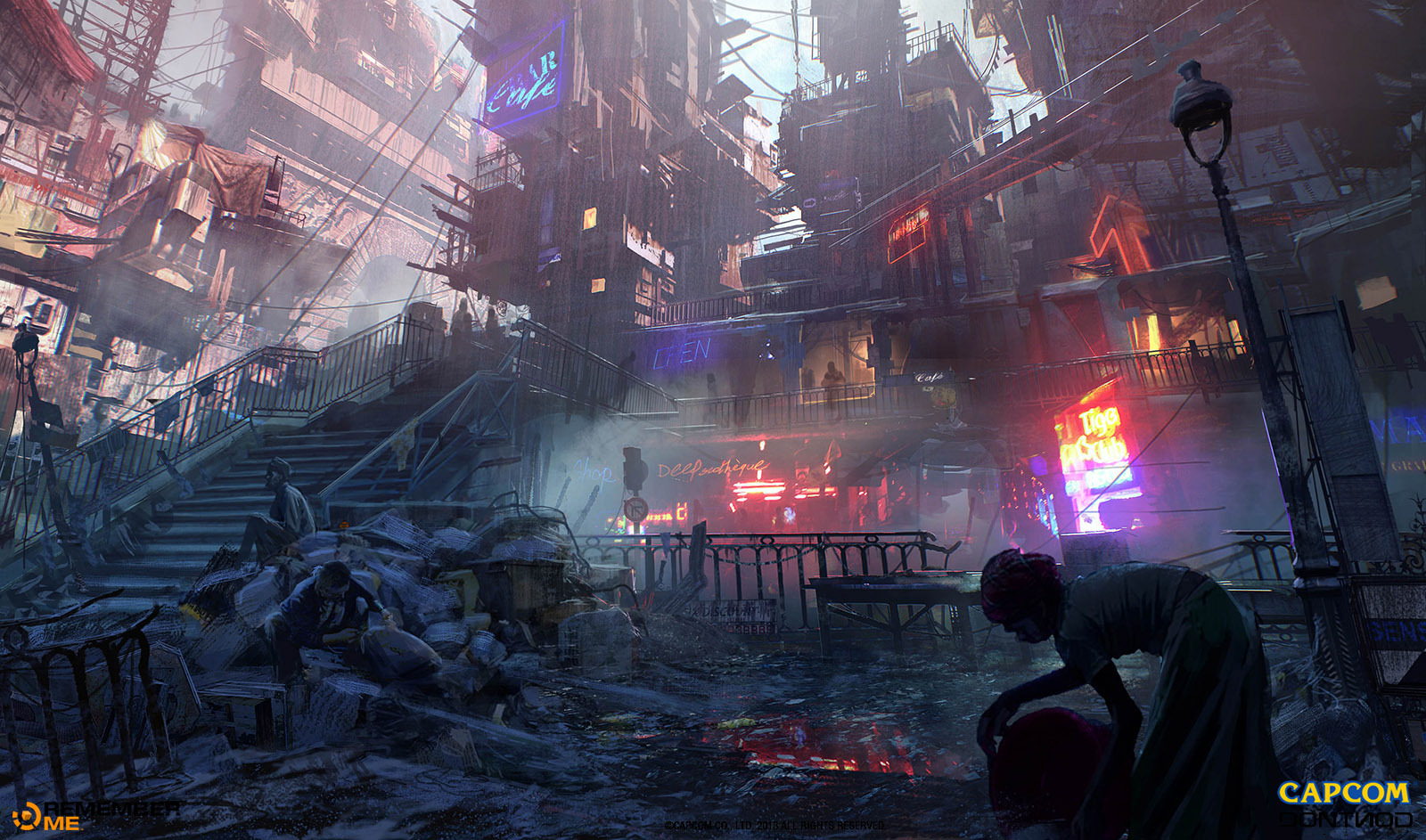The image depicts a highly detailed futuristic cityscape, likely a digital illustration or concept art, possibly connected to the video game company Capcom. The lower right-hand corner features the yellow Capcom logo, hinting at its origin. At the forefront, a woman in a dress is bent over, picking up a round object, and appears as a silhouette due to the intense neon lighting that bathes the city in vibrant hues. Behind her, a street lamp and a brightly lit store complete the scene, with a fence positioned in front of the stores.

The left side of the image is dominated by a large staircase with a handrail, which leads to higher levels of the city. A man sits forlornly on a pile of rubble near these stairs. Above the staircase, there is a construction structure shrouded in smoke and red scaffolding. The city's skyline is filled with jagged brown apartment buildings, featuring numerous balconies, with a prominent blue neon sign that reads "VR Cafe" on one of them. These buildings stretch skyward, casting long shadows and adding to the dark, run-down atmosphere of the lower city, despite the profusion of neon lights and signs illuminating the area. The top right corner reveals a small bridge and a red arrow can be seen behind the street lamp, adding to the intricate and layered design of the futuristic urbanscape.